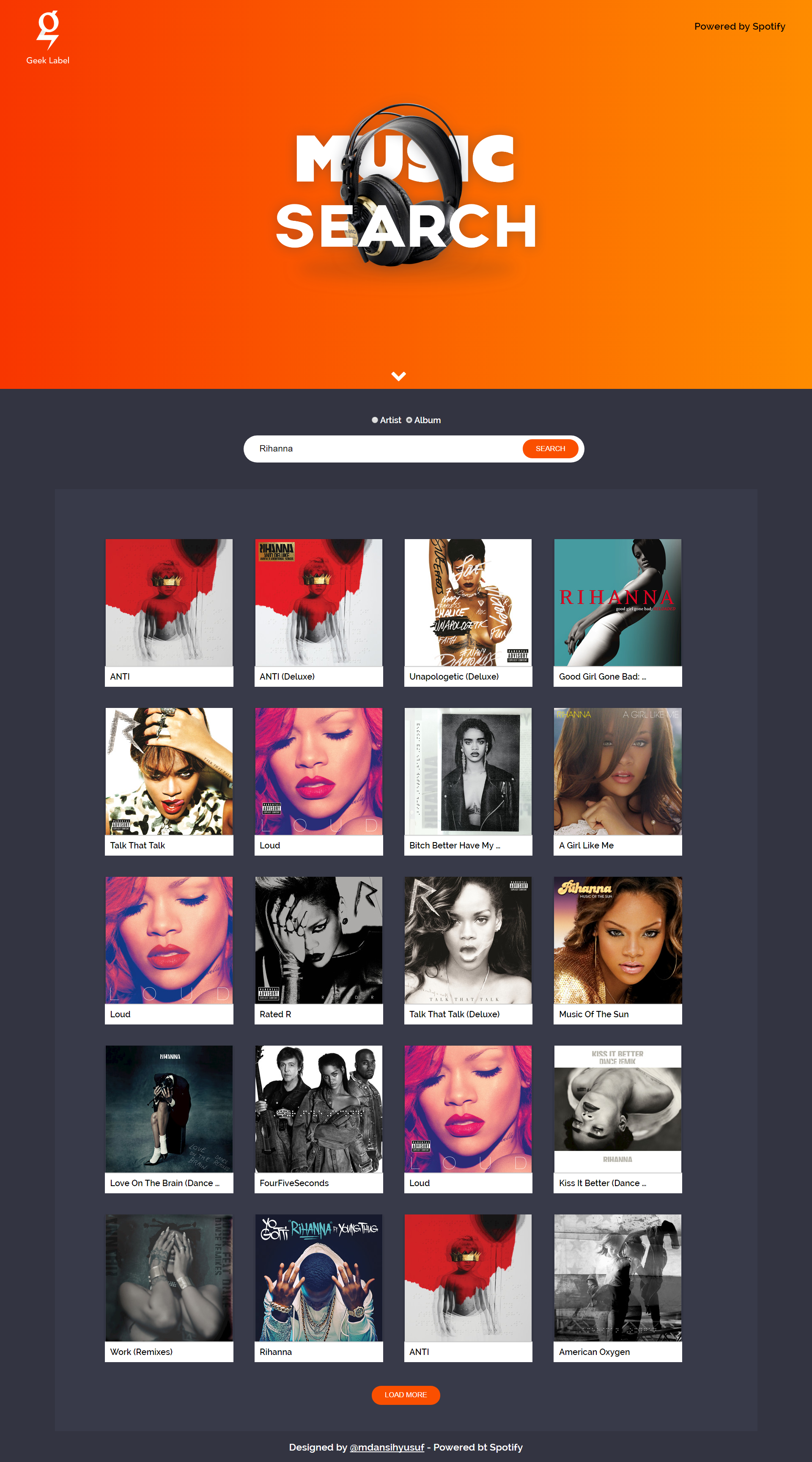This is a highly detailed smartphone screenshot of a webpage from the website "Music Search." The header section features an orange banner with a drop-down arrow on the right side and a logo depicting a pair of headphones. The site indicates that it is "Powered by Spotify."

Below the header is a search bar with the keyword "Rihanna" entered, categorized under "Artist and Album." The search results display several of Rihanna's albums, each accompanied by cover photographs, predominantly showcasing her face. The albums listed include:

- "ANTI" 
- "Unapologetic"
- "Good Girl Gone Bad"
- "Talk That Talk"
- "LOUD"
- "Bitch Better Have My Money"
- "A Girl Like Me"
- "Music of the Sun"
- "Talk That Talk (Deluxe)"
- "Rated R"
- "Love on the Brain"
- "Kiss It Better"
- "Dance"
- "American Oxygen"
- "ANTI (Deluxe)"
- "Work (Remix)"

At the bottom of the search results, there is an additional orange button, though its label is unreadable in the screenshot.